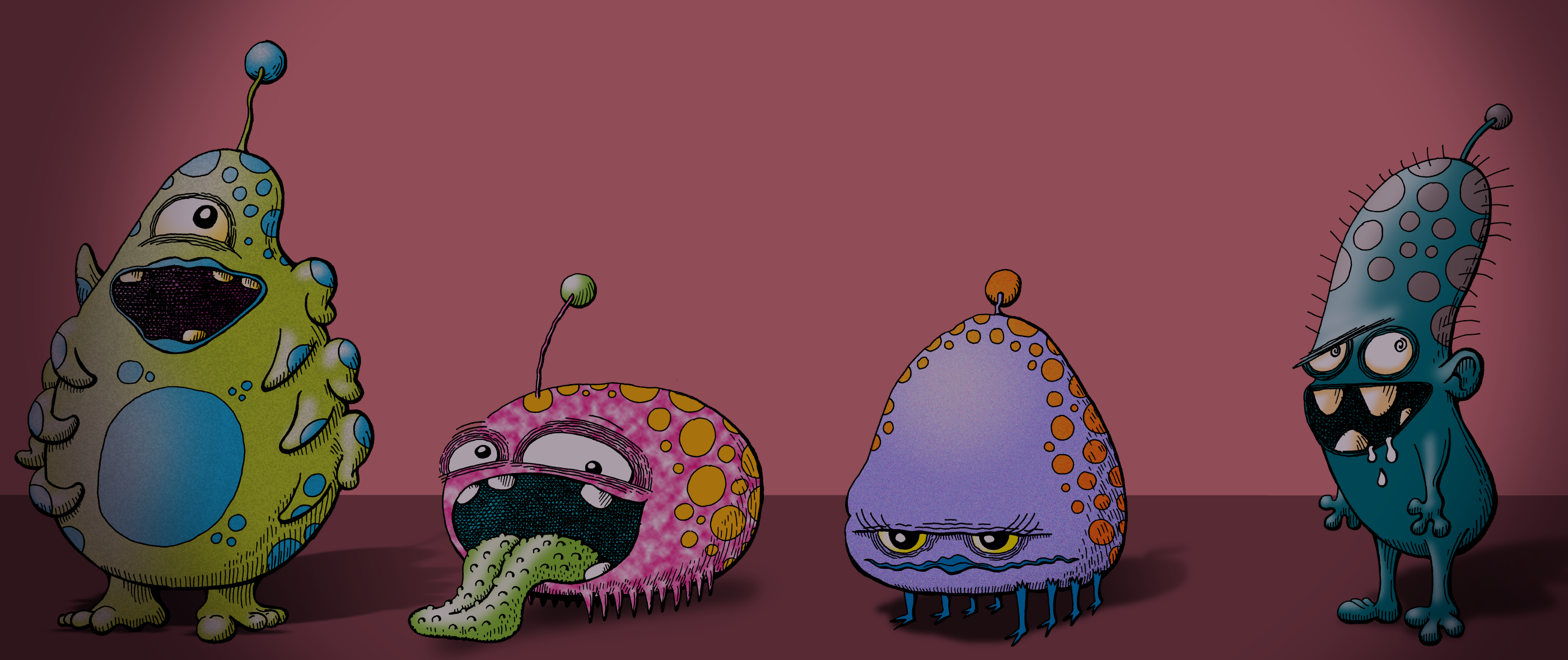The image is a rectangular piece, approximately two inches tall by six inches wide. It depicts four hand-drawn cartoon creatures, potentially representing aliens or viruses, set against a background that transitions from a pinkish-purple tone at the top to a darker purple floor at the bottom.

Starting from the left, the first character is a tall, oblong green creature with blue circles scattered across its body. It has a single eye, a gaping open mouth with four visible teeth, and a skinny antenna on its head topped with a blue ball. This creature stands on two legs.

To its right stands a shorter, round pink creature adorned with yellow or orange spots. It features two eyes, a black open mouth with a protruding green tongue touching the floor, and an antenna with a green ball at the top. This creature has four visible teeth.

The third character is a purple, gumdrop-shaped creature covered with small orange circles. It has two yellowish eyes, long eyelashes, a single unibrow, and a thin blue mouth that is closed. It stands on eight small blue legs and sports an antenna with an orange ball on top.

The final character on the right is a skinny, tall dark green figure with purple dots scattered on its body. It has large white eyes, an open mouth with a hint of drool, and a brownish-pink antenna with a purple ball at the top. This creature stands on two legs and has two arms ending in paws. 

Overall, the unique mix of colors, textures, and quirky anatomical features of these characters creates an interesting visual experience, blurring the lines between digital and traditional colored pencil art.